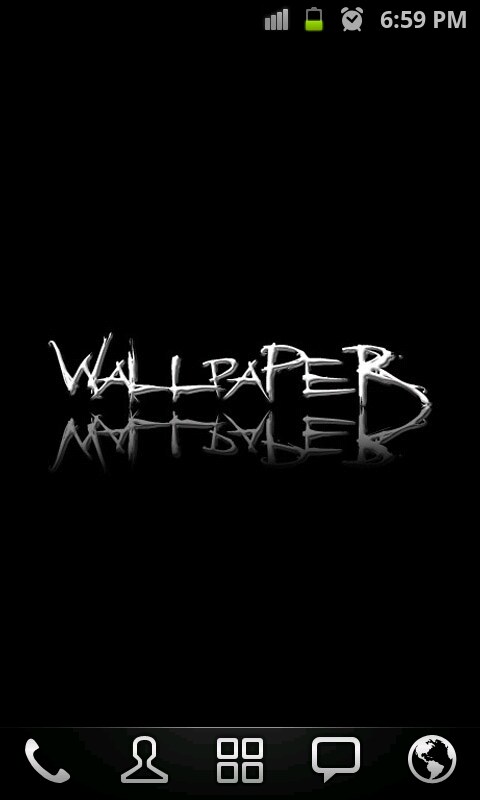This is a screenshot of a smartphone's home screen. The background is entirely black, making the central white text that says "wallpaper" stand out prominently. Below the main text, "wallpaper" is reflected in a faded, mirrored effect, resembling a glossy surface or water. At the top of the screen, the status bar displays the current time, 6:59 PM, alongside usual icons indicating signal strength, battery level—which is about half-charged with some green visible, and an alarm clock symbol. The bottom of the screen features icons for a telephone, contacts, app drawer, messages, and web search. The overall design is minimalist with a stark contrast between the white text and the black background.